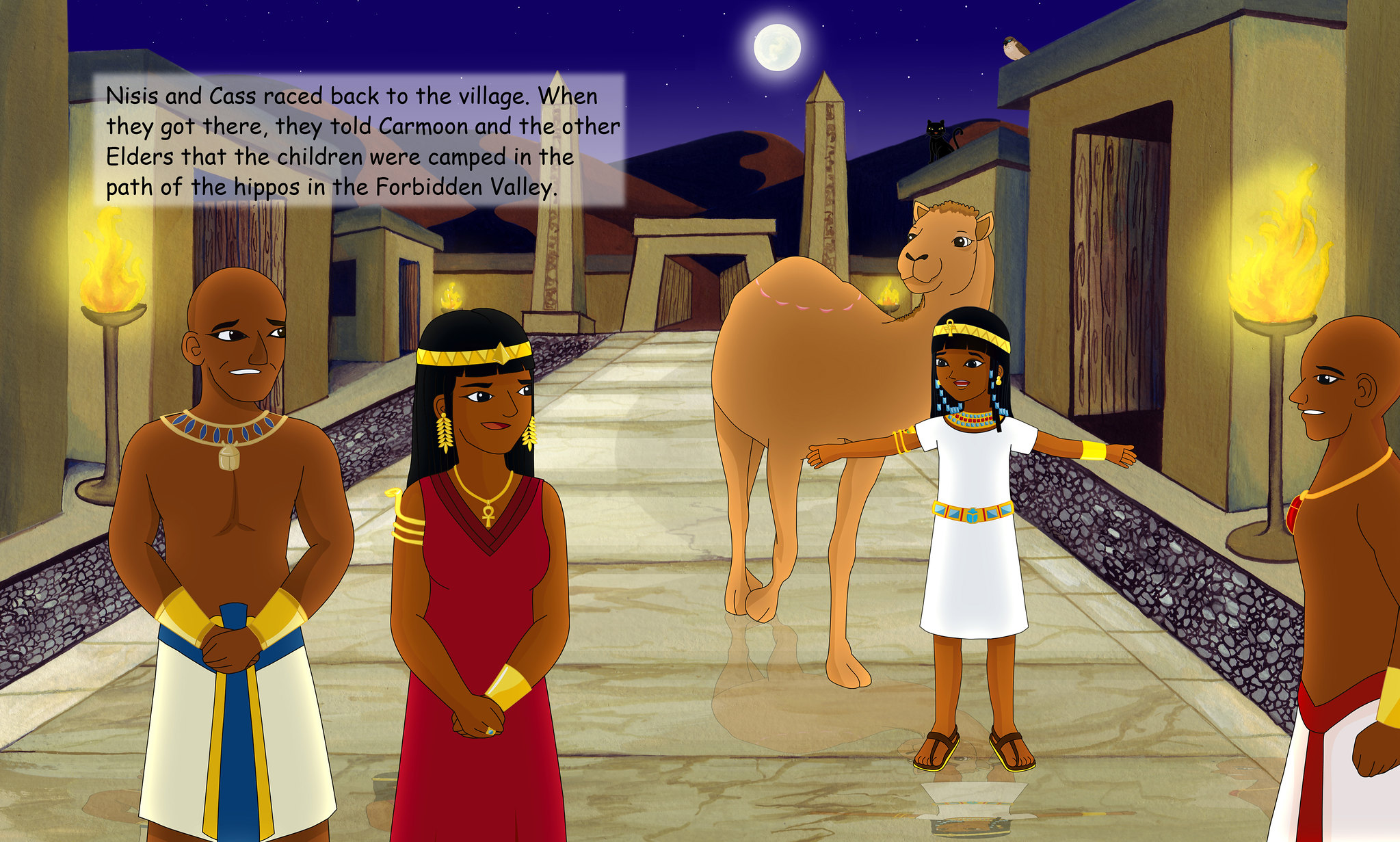The image is a vibrant illustration reminiscent of a children's book, set against the backdrop of a night-time Egyptian scene. Dominating the background are obelisks and pyramids silhouetted against the purple night sky, which is illuminated by a bright moon. Sand dunes stretch out, adding to the mystic ambience. Atop a house perched a cat and a bird, adding subtle life to the scene. The distant fires blazing in tall, metal vase-like stands also highlight the setting.

In the foreground stands a young girl garbed in traditional Egyptian attire, adorned with gold earrings. She is positioned in front of a tan camel, accentuating the scene's authenticity. To her left is a shirtless man also dressed in Egyptian clothing, including a white and blue skirt, gold accessories, and a collar. To her right, a couple clad in Egyptian attire make an impression; the woman in a red dress and the shirtless man in a white, blue, and gold skirt. Their regal appearance suggests nobility or royalty. The narrative derived from the image hints at a story where characters named Nysus and Cass inform Karmun and the elders about the children camped in the path of hippos in the Forbidden Valley, enriching the scene with an adventurous undertone.